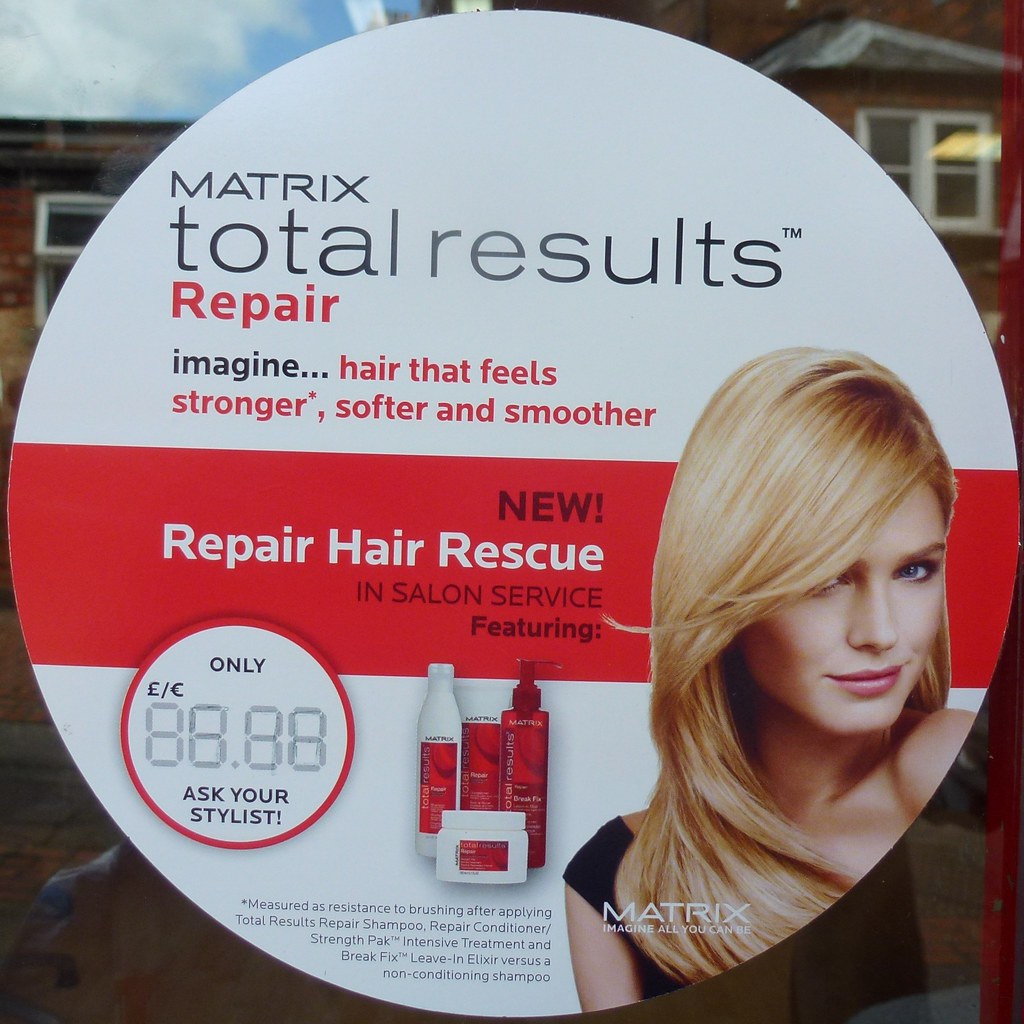A large circular sticker advertisement is affixed to a window, prominently displaying reflections of a building from across the street. The predominantly white background of the circle contrasts with a striking red banner running horizontally through its center. At the top of the circle, black text reads, "Matrix Total Results Repair. Imagine hair that feels stronger, softer, and smoother." Positioned in front of the red banner is a blonde woman with shoulder-length hair partially covering her eyes, giving a seductive look. Her hair features the text "Matrix. Imagine all you can be." Below this, the red banner proclaims, "New Repair Hair Rescue and Salon Service Featuring."

The lower portion of the sticker showcases images of several Matrix hair care products, including three bottles and a small jar. Adjacent to these images is a placeholder for pricing, marked with the text, "Only – Ask Your Stylist," though no specific price has been set. The overall impression is of a high-quality hair care product advertisement, likely situated at a salon window, with the reflective surface providing an intriguing glimpse of the urban environment beyond.